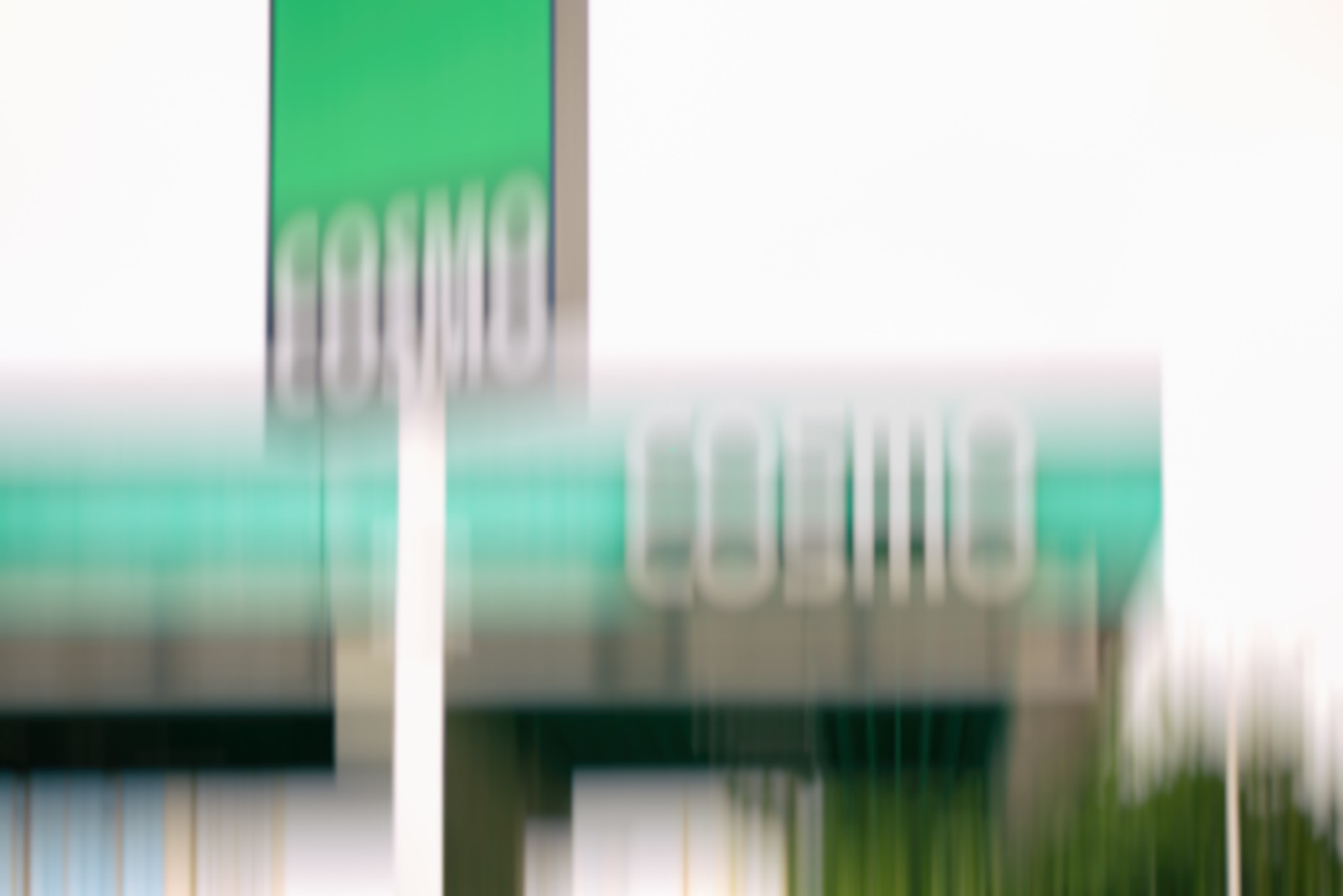This blurry photograph captures a storefront, identifiable by a high-mounted sign on a white post. The sign features a green background with the word "Cosmo" written in white lettering at the bottom. The storefront itself has a matching green stripe at the top, also seemingly inscribed with the word "Cosmo," though the text is hard to discern due to the blurriness. The remainder of the building is gray, and the sky overhead appears white, likely due to overcast weather or overexposure in the photograph. Towards the bottom of the image, several pillars supporting the outer facade of the building are visible.